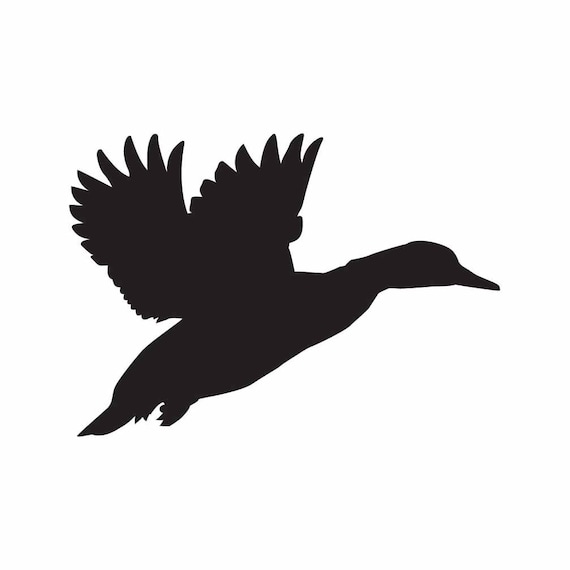The image showcases a detailed silhouette of a duck in mid-flight against a stark white background. The duck is entirely black, facing to the right with its rounded head and beak clearly outlined. The head is positioned straight, while the slender body angles from the top right towards the bottom left. Both extended wings are visible behind the duck's back, appearing mid-flap with distinct feathers that fan out, showcasing intricate details. The tail, short and tucked feet with visible talons, add to the realism of the silhouette. The wings are notably large compared to the body and feature prominent primary feathers with multiple segments. The overall composition emphasizes the elegance and motion of the duck in flight, despite the image's minimalistic color scheme.